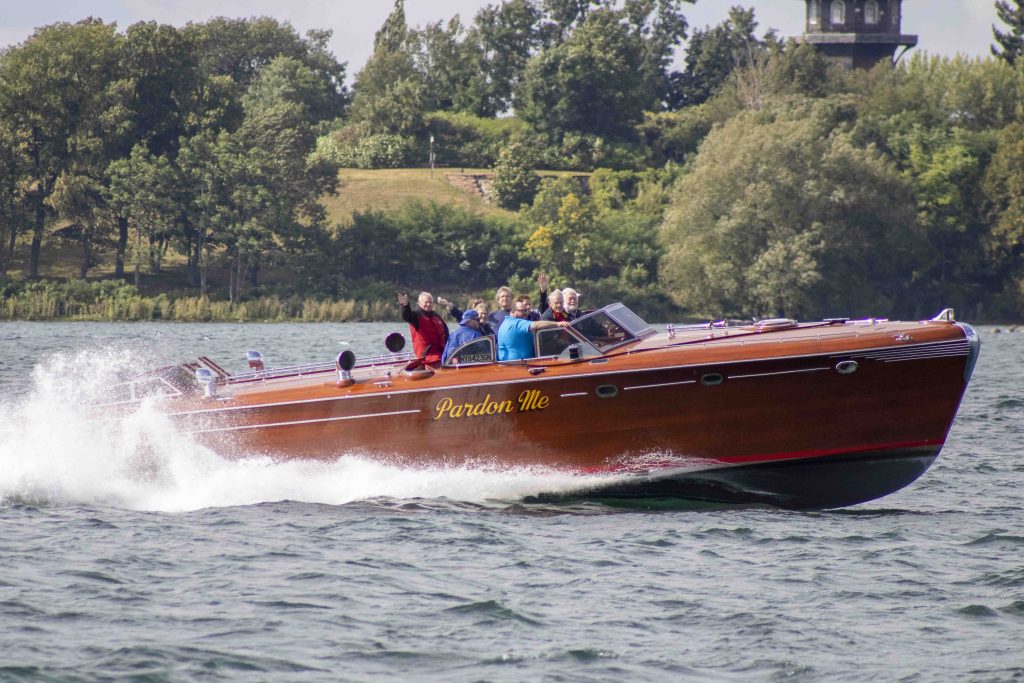This vibrant color photograph captures eight older Caucasian men enjoying a ride on a classic wooden speedboat, reminiscent of a Chris-Craft style vessel. The boat, named "Pardon Me" as indicated by its golden cursive text on the side, features a deep brown varnished wooden hull complemented with a black bottom and a red stripe, and a low-standing glass windshield at the center. The boat is seen cutting through the greenish-blue water at high speed, creating large splashes and a frothy white wake behind it. Several of the men are cheerfully waving towards the camera, which seems to be either from another boat or the shore. They are dressed in various colors, including red, blue, and black tops, signifying an atmosphere of joy and camaraderie. In the background, a gentle hill carpeted with green grass, possibly part of a golf course, rises up, adorned with tall, lush trees under a clear blue sky. The scene is a picturesque moment of leisure and enjoyment on the water.